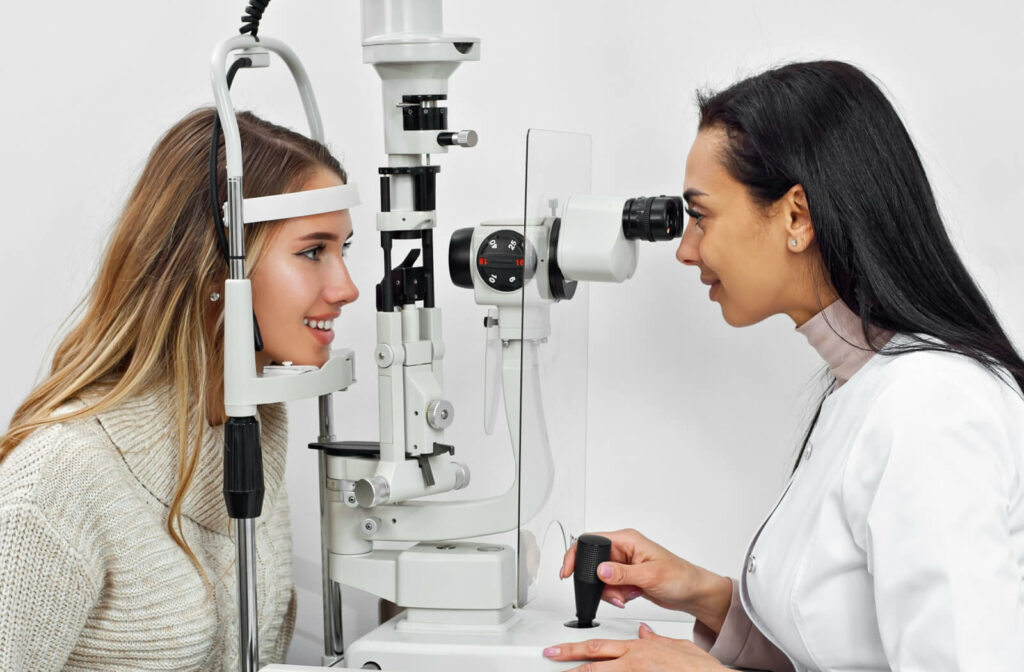The image captures a detailed scene at an eye doctor's office. On the left side sits a young white woman, estimated to be around 18 or 19 years old, with long, blondish-brown hair featuring darker roots. She is smiling and resting her head in a specialized device designed to limit movement during the eye examination. The young woman is dressed in a light-colored, wool-like sweater, possibly white or light brown, and she sports small diamond earrings.

Opposite her, on the right, stands the eye doctor, a lighter-skinned woman with black hair, who is focused on examining the patient's eyes through a sophisticated black-and-white technical instrument. The doctor is wearing a white lab coat over a light pink or beige turtleneck and has small stud earrings and pink nail polish. Her hand is engaged with a joystick on the instrument, adjusting the settings and controlling the eye examination procedure. The composition and interaction between the patient and the doctor, along with the detailed descriptions of their attire and the apparatus, create a precise and vivid portrayal of an optometry exam.